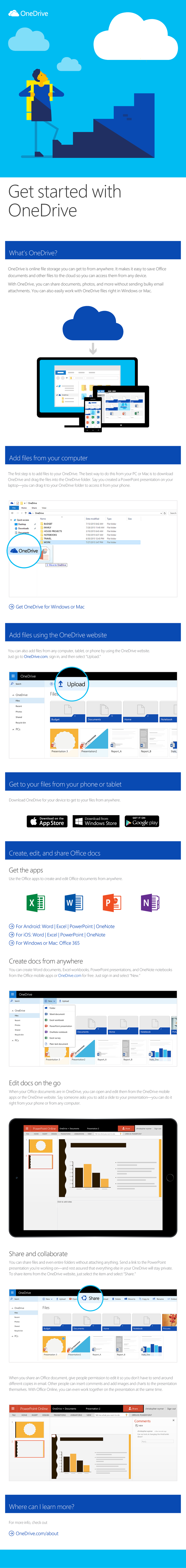**Screenshot of OneDrive Introduction Page**

The screenshot is a vertical and narrow image, possibly from a website or an app. The top features two puffy clouds with a smaller one in front, the background showcasing larger clouds in light blue. In the center, a thin white font spells "OneDrive" against a baby blue sky. 

Prominently displayed near the top right, a graphic of a stick figure person with black hair, wearing a yellow backpack and a blue shirt that fades from light to dark blue, walks up a set of blue stairs that transition from dark blue to light blue. This illustration appears to be crafted by a graphic artist or AI.

Below this illustration, on a white background with thin black text, the heading reads, "Get started with OneDrive," with "OneDrive" in uppercase and lowercase letters. A blue rectangular banner towards the bottom contains the text "What's OneDrive?" in white font. Below this banner, in smaller gray font, a brief explanation of OneDrive is provided, accompanied by an image featuring a blue cloud with a gray arrow pointing down towards a monitor and a smartphone.

Separating the sections, a blue banner spans from left to right with white font saying, "Add files from your computer." Below, it displays a Windows explorer window with various folder icons and an enlarged, circled "OneDrive" option.

Another thin line beneath this section leads to a small light blue font reading, "Get OneDrive for Windows or Mac," next to a circle with an arrow pointing to the right.

The next section's white background features another blue banner with white text, "Add files using the OneDrive website." Below, an illustration of a Windows window showcases an "Upload" button, marked by a light blue circle with an arrow pointing up and a blue line underneath it.

Moving down, a blue banner states, "Get to your files from the phone or tablet," with icons depicting options to download from the Apple App Store, Windows Store, and Google Play.

Another banner follows with the text, "Create, edit, and share Office Docs," leading into a section labeled "Get the apps." This part showcases four colorful folder icons: green with a white X, blue with a white W, orange with a white P, and purple with a white N. Beneath, it states, "Create Docs from anywhere," illustrating a Windows explorer interface for document creation.

The last section within the screenshot, labeled "Edit Docs on the go," features a close-up of a tablet displaying graphs in blue and tan colors. A subsequent section titled "Share and collaborate" includes a schematic for document sharing. Finally, the bottom of the page suggests visiting "OneDrive.com/about" for more information, marked by a circular icon with an arrow.